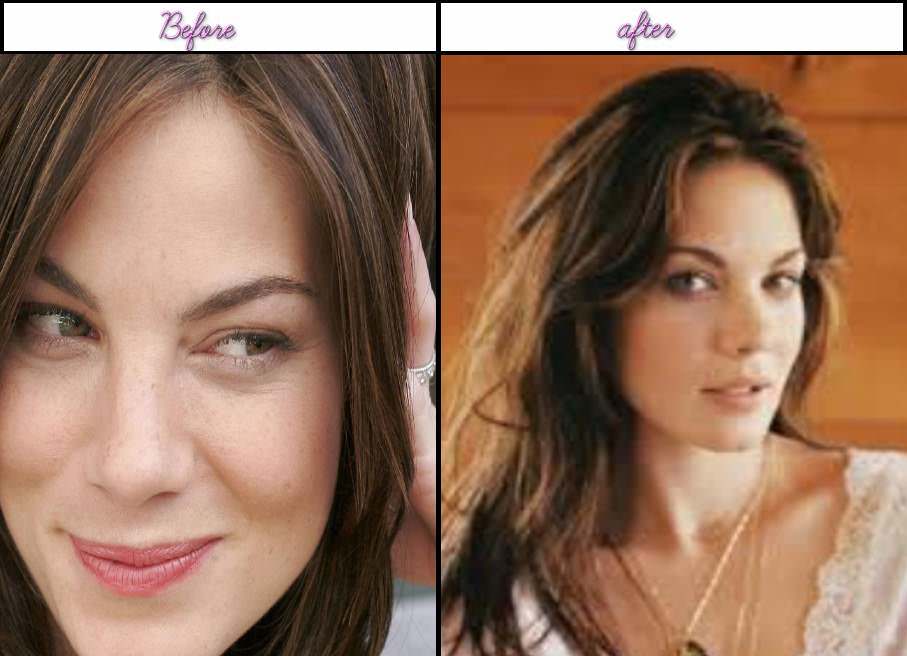This horizontally aligned rectangular image showcases a dramatic transformation through a "before and after" layout. The photo is split into two vertically aligned rectangular sections. 

On the left, the "before" section is labeled with the word "before" in elegant purple cursive against a pristine white background. It features a close-up shot of a woman’s face. She has a warm smile with her mouth closed and wears pink lipstick. Her eyes, possibly green or brown, gaze gently at the camera, and she has straight brown hair framing her face.

Contrastingly, the "after" section on the right is marked with "after," also in purple cursive letters, set against a white background. This image reveals more of the woman's upper body. Her hair is now styled in soft waves, cascading over her right shoulder, and she wears a fashionable white top with delicate lace trim. Her transformation is accentuated by her radiant smile, this time showcasing her teeth. A gold necklace graces her neck, adding a touch of elegance. The background in the "after" photo is a warm brown, providing a cozy and inviting atmosphere, unlike the indiscernible background in the "before" image.